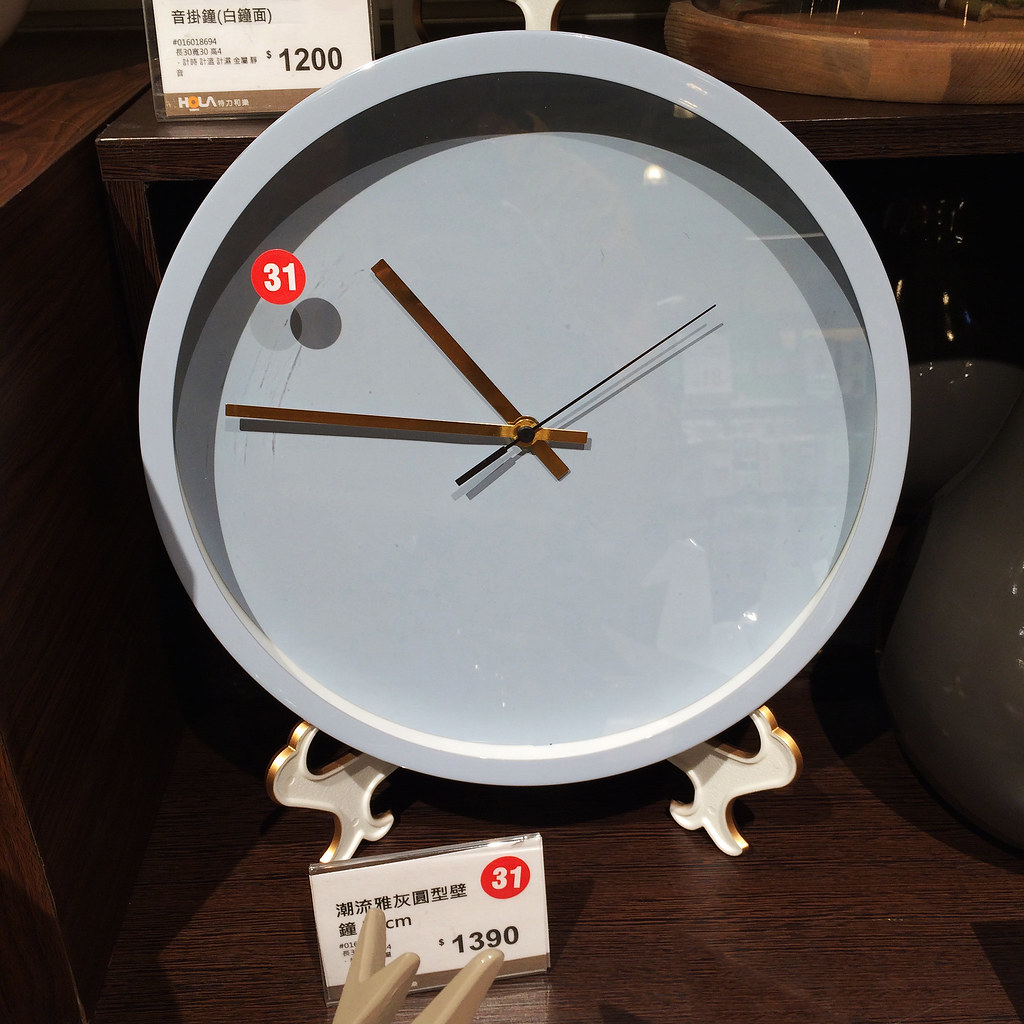This photograph captures a close-up view of a store display featuring a large, round, light teal clock situated on a wooden surface. The clock boasts white decorative feet and a face covered by a transparent plastic or glass lens. Adorning the clock face is a prominent red sticker with the number "31" in white. Notably, the clock face is devoid of any numerical markings or dashes, showcasing a minimalist design with just three hands – two brown and one black. In front of the clock, resting on the wooden surface, is a small white card displaying the price "1390" along with some Asian script. A striking red circle housing the white number "31" is also printed on the card, ensuring that all price-related information complements the clock's aesthetic appeal.